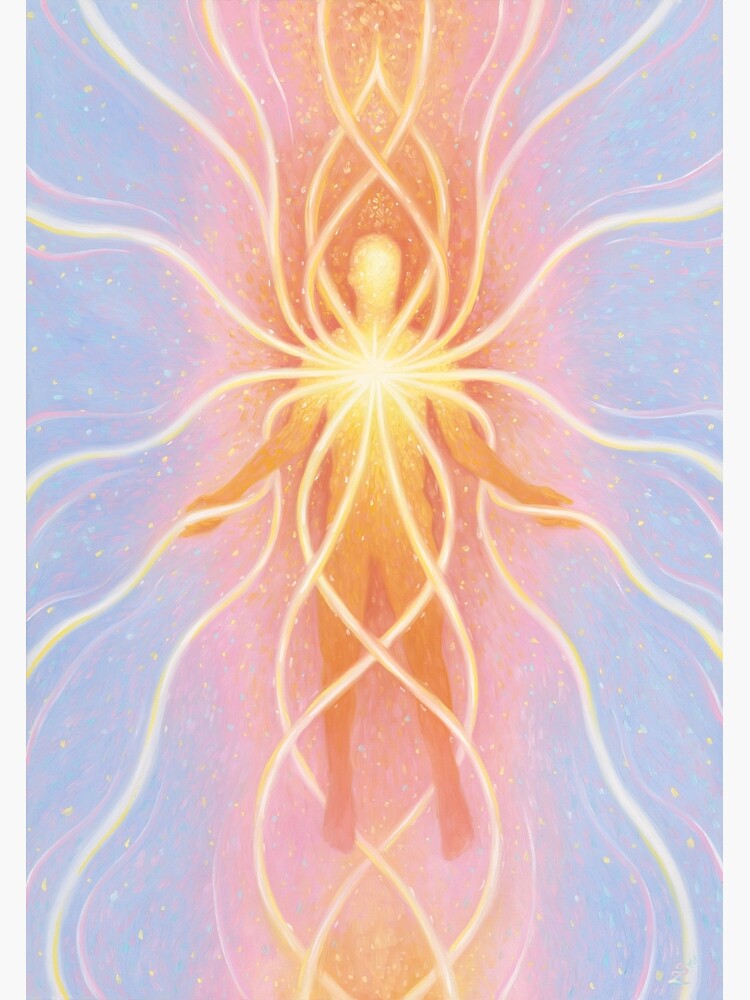The image depicts a striking, abstract figure of a man prominently centered against a vibrant background. The man, rendered in shades of yellow and orange, lacks distinguishing facial features but is distinguished by the intense hues of his body: yellow from the head through to the upper torso transitioning to orange across the lower arms, abdomen, and legs. Energetic waves emanate from his chest in all directions—top, left, right, and bottom—painted in vivid yellow and snake-like in appearance. These waves create an impression of the figure being illuminated or engulfed in radiant light. Surrounding the figure, the background shifts from orange directly behind him to pink, with the outer edges infused with blue and peppered with tiny dots of blue, yellow, and pink. This compelling composition gives the sense of the figure floating, infused with and emitting an ethereal energy, painting an evocative image of a space being or an energy man.